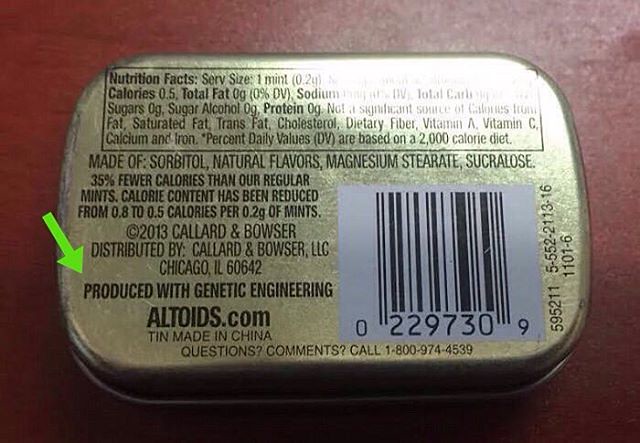This is a detailed photograph of the back of a gold-colored Altoids mint tin. The back of the tin features a large black and white barcode and a prominent Nutrition Facts label in black font. The ingredients listed include sorbitol, natural flavors, magnesium stearate, and sucralose, with a note stating that the mints have 35% fewer calories than regular mints, reducing calorie content from 0.8 to 0.5 calories per 0.2 grams of mints. A green arrow highlights the phrase "produced with genetic engineering," and there is a bold statement noting that the product is made in China. Further information includes a copyright date of 2013, attributed to Callard and Bowser, LLC, distributed from Chicago, Illinois, 60642. Additionally, there is a phone number for questions or comments (1-800-974-4539) and a website (altoids.com). The tin rests on a brown table, and parts of the text are obscured by a bright light shining on the right side.